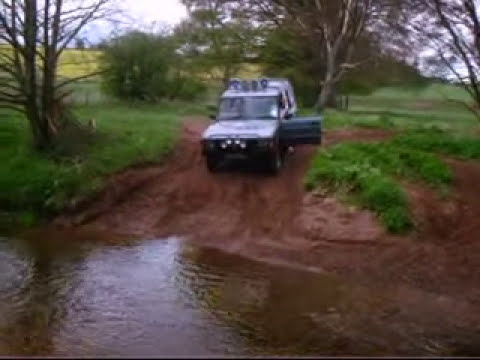This detailed photograph captures a rural, outdoor setting during daytime. The scene features a shallow, brown creek in the foreground, bordered by a dirt embankment. A gray or metallic-colored Jeep, equipped with roof lights and lights on the front, is prominently positioned on a dirt road in the center of the image. The Jeep's driver's side door is open, suggesting it has just stopped, and there are visible tire marks on the dirt road leading to the water's edge. The image is filled with lush green grass flanking the dirt road and a backdrop of abundant trees and bushes, under a clear white and blue sky. The overall palette includes shades of brown, beige, green, dark green, white, silver, gray, light blue, light green, and black. Despite the somewhat blurry capture, the photograph effectively conveys the serene and natural environment of a rural area with a focus on a solitary Jeep, seemingly on an adventurous exploration towards the creek.